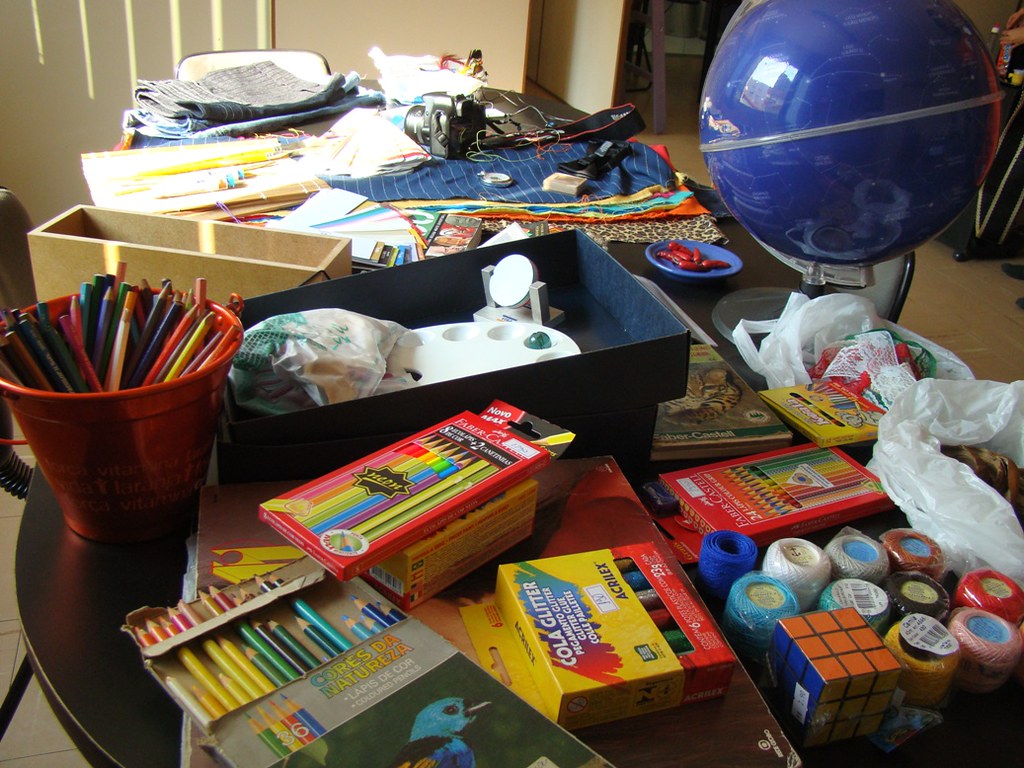The photograph showcases a sprawling brown craft table, evidently set up for children's art activities. The table, quite long in appearance, is littered with an assortment of creative supplies. Dominating the table's top right corner is a sizeable dark blue globe. To the top left, a glimpse of a descending staircase and part of its guardrail is visible.

On the table's surface, at the bottom, several packs of colored pencils and an assortment of markers can be clearly seen. To the bottom right rests a collection of paint jars, next to which stands a fully solved Rubik's Cube, displaying its orange, blue, and yellow faces. To the left, a set of colored pencils is gathered in a red pot. Scattered across the table's top, various knitting materials and pieces of cloth in different colors add to the vibrant array of supplies. The scene is an inviting chaos of creativity, ready for young artists to explore.